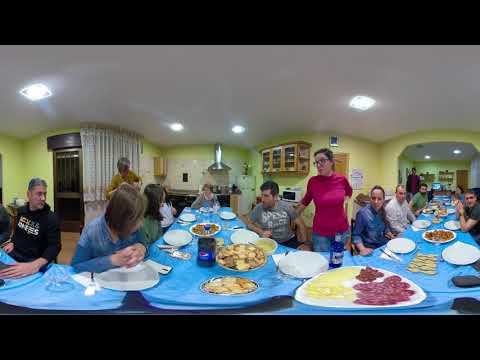This image features an indoor panoramic view of an expansive dining setup. The setting appears to be a large kitchen or dining area, possibly in a home or a restaurant, characterized by three long tables draped with light blue tablecloths extending into the distance. Each table is neatly set with white plates, silverware, and white napkins, indicating an imminent meal. The tables are adorned with various food platters, including what seems to be pastries, pepperoni slices, and cheese, though some of the items are not clearly identifiable. 

People of mixed genders and ages, casually dressed, are seated along both sides of the tables, engaged in different activities, suggesting a relaxed and communal atmosphere. The background shows yellowish-green walls with wood cabinetry, a door to the left, a window area with curtains, and a kitchen area visible in the middle distance, complete with a refrigerator, stove, and vent hood. The ceiling is white, featuring recessed lighting. A possible sheet of thread is noted on the lower right, hinting at additional activities or decoration. The scene exudes a warm and convivial vibe, emphasizing the shared experience of a communal meal.